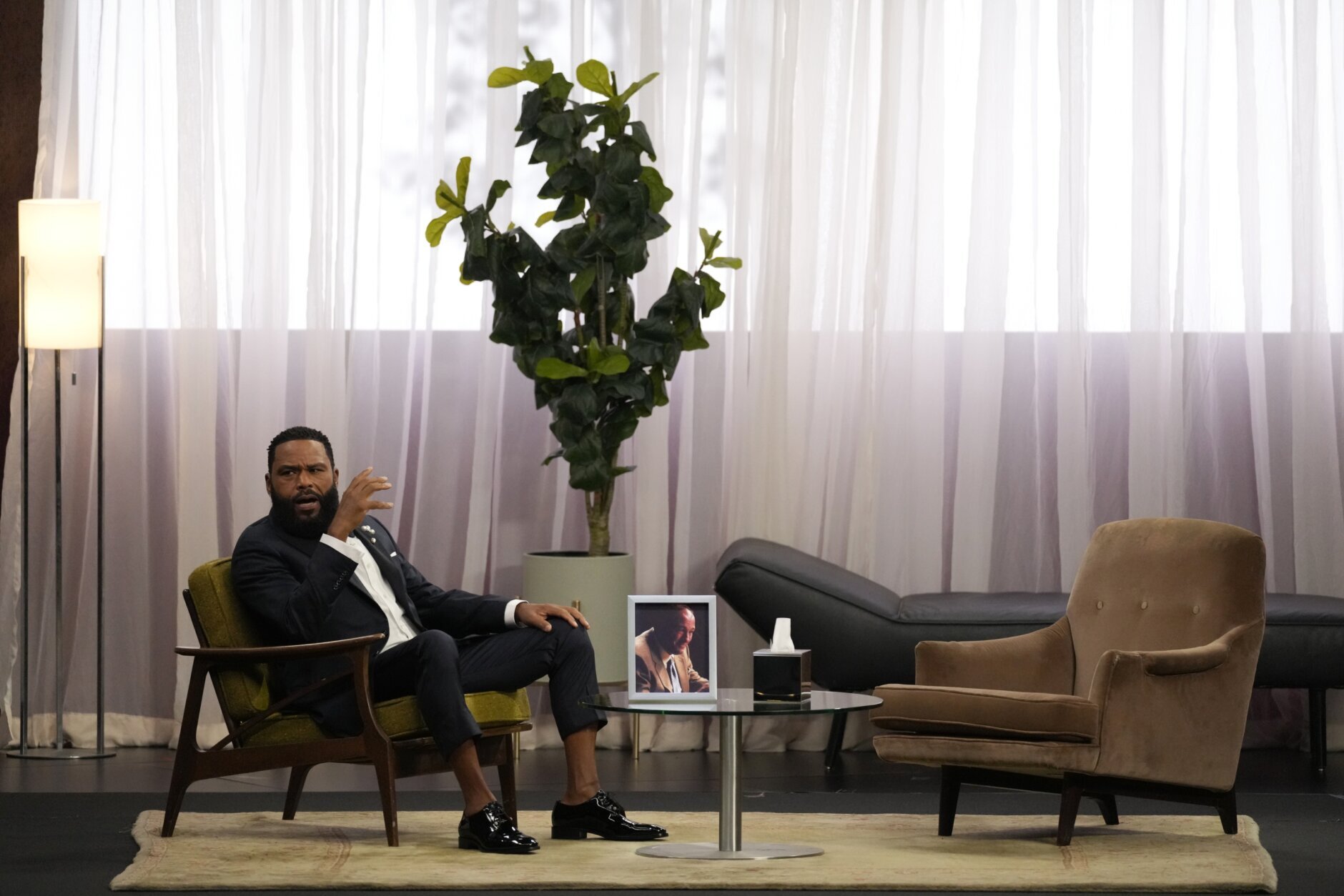The image depicts a well-dressed black man, possibly actor Anthony Anderson, in a modern mid-century styled living room. He is seated in a low, wooden-framed chair with olive green cushions, wearing black slacks, a black jacket, shiny black leather shoes, and a white button-up shirt. His black pants are slightly rolled up, and he has a beard. He is engaged in conversation, gesticulating with his right hand while his left hand rests on his knee.

The surroundings feature a polished gray concrete floor with a cream-colored area rug under his chair. A low round coffee table, perhaps made of shiny stainless steel with a glass top, stands in front of him, holding a box of tissues and a framed photo, possibly of Michael Jordan. Opposite him is an unoccupied high-back upholstered armchair in light tan suede. 

The backdrop is a large lateral window that spans the width of the photo, draped with sheer white curtains allowing natural light to filter in. A tall potted plant stands in front of the window, reaching about five feet in height. To the left of the man, a tall floor lamp with a barrel-shaped shade and a pull chain is lit, casting a warm glow. A long, gray-upholstered bench, reminiscent of a classic psychiatrist's chaise lounge, is positioned nearby, further enhancing the room's mid-century modern ambiance.